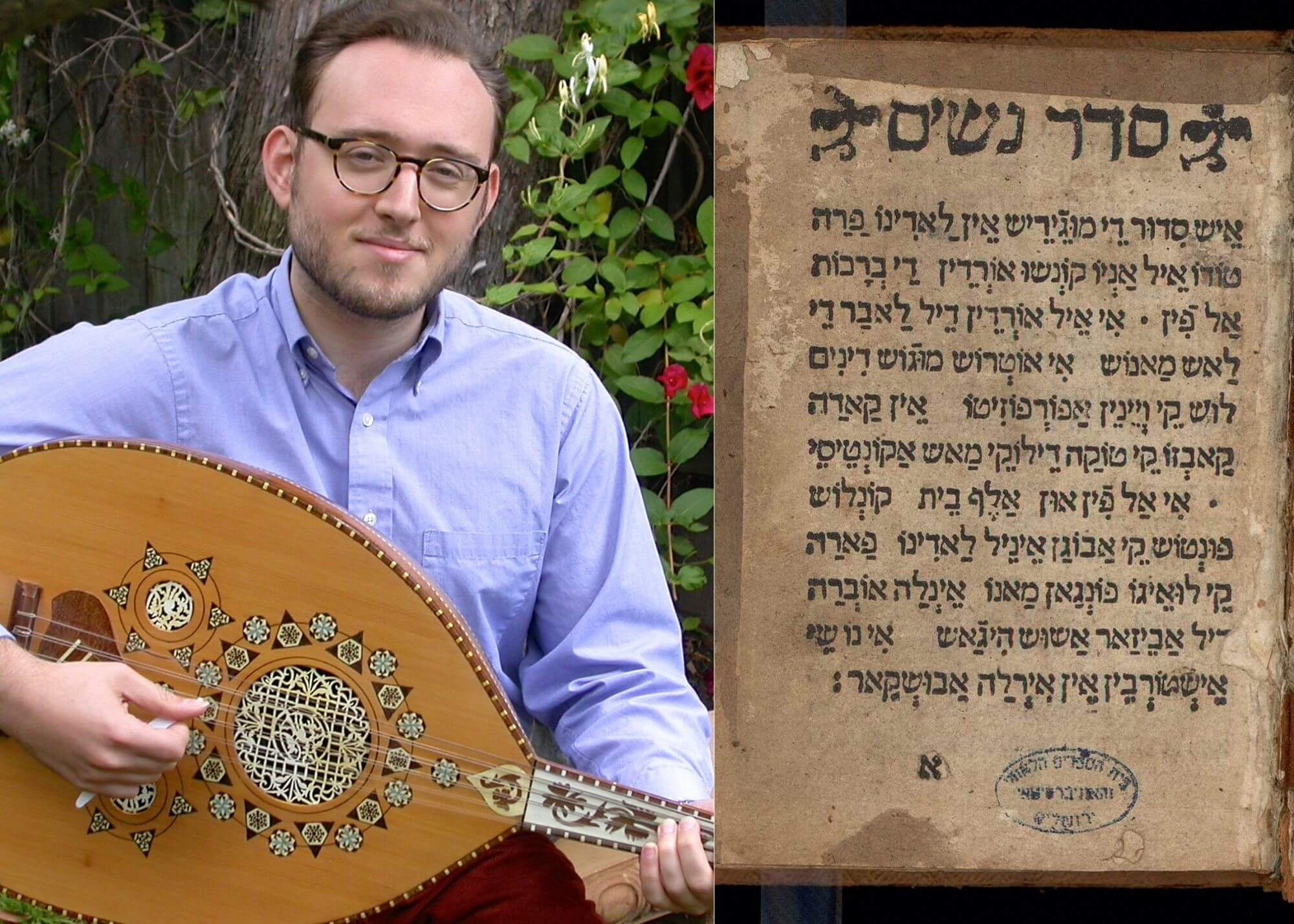The image features a light-skinned man with short brown hair, a close-shaven beard, and black-rimmed horn glasses, smiling slightly while seated in front of a flowering bush with green leaves and red flowers. He is wearing a blue button-down shirt with a collar and is holding a tan, stringed instrument that resembles a cross between a ukulele and a banjo. This instrument is decorated with white triangular floral patterns in a stained glass or mosaic style, and it has a headstock adorned with brownish vine-like designs. The man is playing the instrument with his right hand, and beside him is an upside-down sign or document with ancient-looking text written in a foreign language, possibly Hebrew, appearing to be drafted on stone.